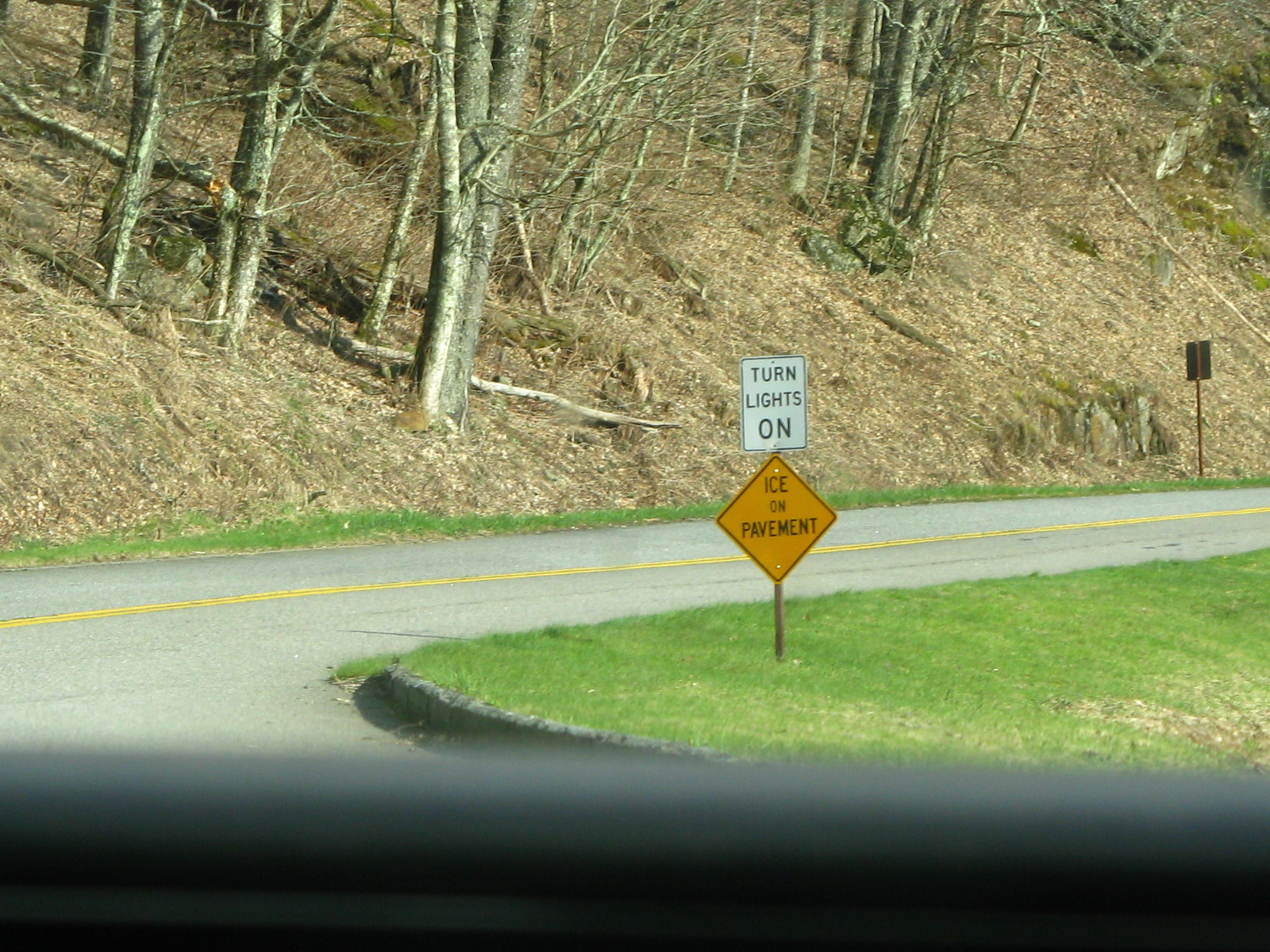This meticulously detailed image captures a forest landscape during a leafless season, characterized by a road running in front of it. The photograph appears to have been taken from inside a vehicle, evidenced by a blurry, black lower edge that seems to be part of the car's interior. The road, featuring two lanes separated by a double solid yellow line, winds to the right. 

On the right side of the image, there is a broad grassy patch, and prominently displayed within this area is a yellow diamond-shaped sign with "Ice on Pavement" written in black letters. Directly above this, a white rectangular sign instructs drivers to "Turn Lights On." The grassy patch is bordered by a curb that curves and possibly leads to a parking lot or side street. On the left side of the road lies another grassy strip, beyond which a hill rises, covered with dead grass and leafless trees. The overall atmosphere suggests a cold season, likely late autumn or winter, contributing to the stark nakedness of the trees in the forest.